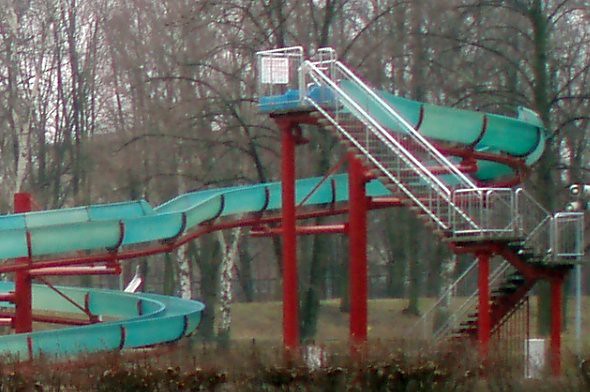The image captures an old and abandoned water slide in what appears to be a deserted amusement park or playground. The slide, which is a blend of aqua green and bluish-green hues, snakes around with multiple levels before eventually dropping to the bottom. Supporting the slide is a series of red-painted metal posts and railings, adding a stark contrast to the otherwise muted scene. The stairway to the slide entry consists of two sets of steps with a flat platform in between, also painted red. Surrounding the slide is a backdrop of bare trees, suggesting the image was taken either in late fall or early spring, as no leaves are visible and the sky peeks through the branches. The entire area, set in a grassy field, exudes a sense of abandonment, with no people present, further emphasized by the worn and unused appearance of the water slide.